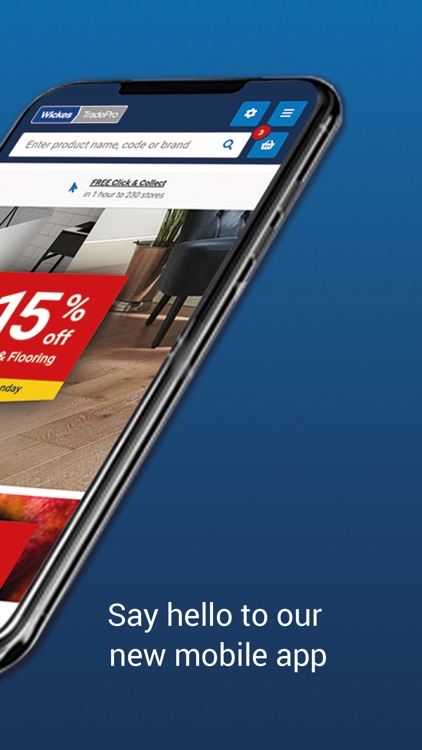**Detailed Caption for App Advertisement Image:**

The advertisement image is designed with a blue gradient background, transitioning from medium blue at the top to a darker blue at the lower right-hand corner. The focal point of the image is a smartphone, positioned in a rotated manner with its lower left quarter cut off by the edge of the image. 

Displayed on the smartphone screen is a well-furnished room featuring a stylish chair, flooring, and a potted plant, emphasizing the interior design aspect. Additionally, there is a coupon depicted on the screen, offering a 15% discount on flooring services. 

In the central, lower right section of the image, just below and to the right of the smartphone, there is a white text message that reads, "Say hello to our new mobile app." This slogan indicates the introduction of a new mobile application, presumably related to the services advertised.

The upper left-hand corner of the smartphone screen displays the text "WICKES Trader Pro," which may refer to either the name of the company or the app itself. This advertisement aims to promote the mobile accessibility of the company's products or services, likely related to flooring and interior design.